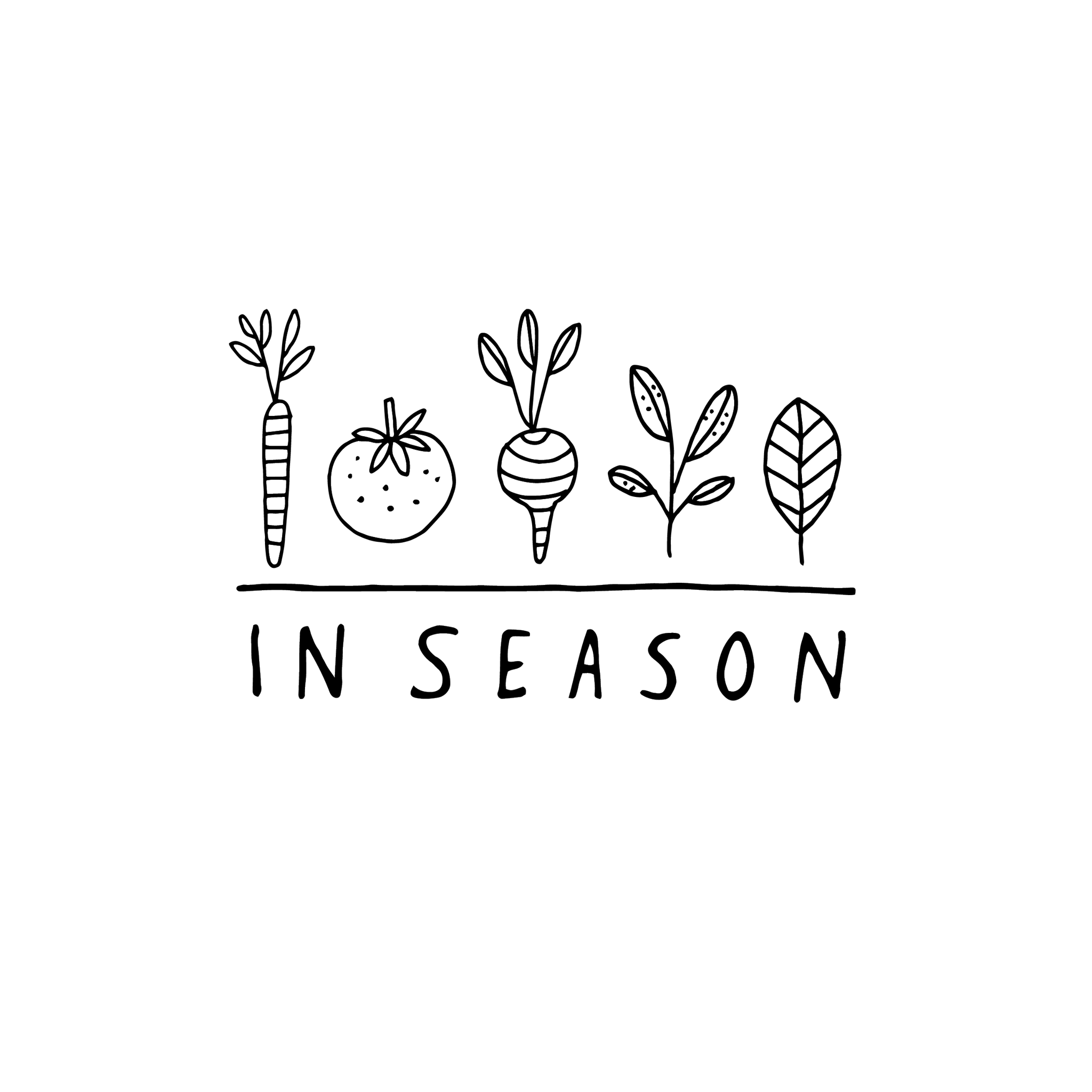This is a horizontally-aligned hand-drawn graphic, black on a white background with no defined borders. At the bottom, in large, all-capital letters, it says "IN SEASON.” Directly above this text is a thin, solid black line. Positioned above the line are five hand-drawn illustrations of various plants and vegetables arranged from left to right. The first drawing depicts a carrot, identifiable by its vertical segments and simple leaves at the top. Next to the carrot is a fruit, likely a spotted strawberry or tomato, characterized by its dotted texture and a star-shaped set of leaves at the top. The third illustration is possibly a beet, with curved, horizontal stripes and simple leaves emanating from the top. Following that is a plant with a stem bearing four leaves, each leaf detailed with veins and spots. The final illustration on the right is a single, solid leaf, featuring a central vein with smaller veins branching off symmetrically. The overall aesthetic of the graphic conveys a handcrafted and rustic charm, suggesting that it might be promotional artwork for a local or roadside market, likely in the United States.